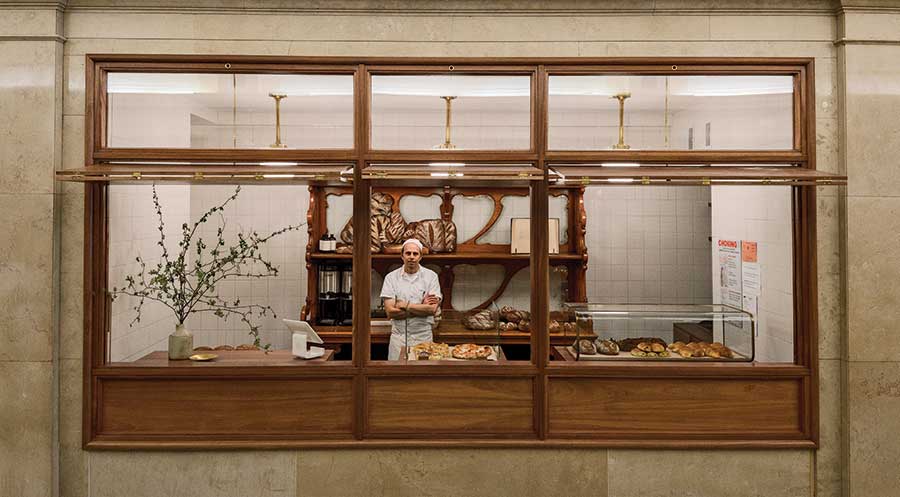The image depicts the interior of a bakery as seen through a rectangular window with three partitions and glass panels. In the center of the scene, a baker dressed in all white, including a white cap, stands with arms crossed. To the right, a display shelf houses a variety of baked goods such as croissants and other pastries, clearly visible through a protective glass case. A brown table holds a white stand, presumably for displaying more items. To the left, a potted plant with vibrant green leaves in a white vase adds a touch of nature. The background features shelves and a few posters on the wall, enhancing the cozy and authentic baking ambiance.